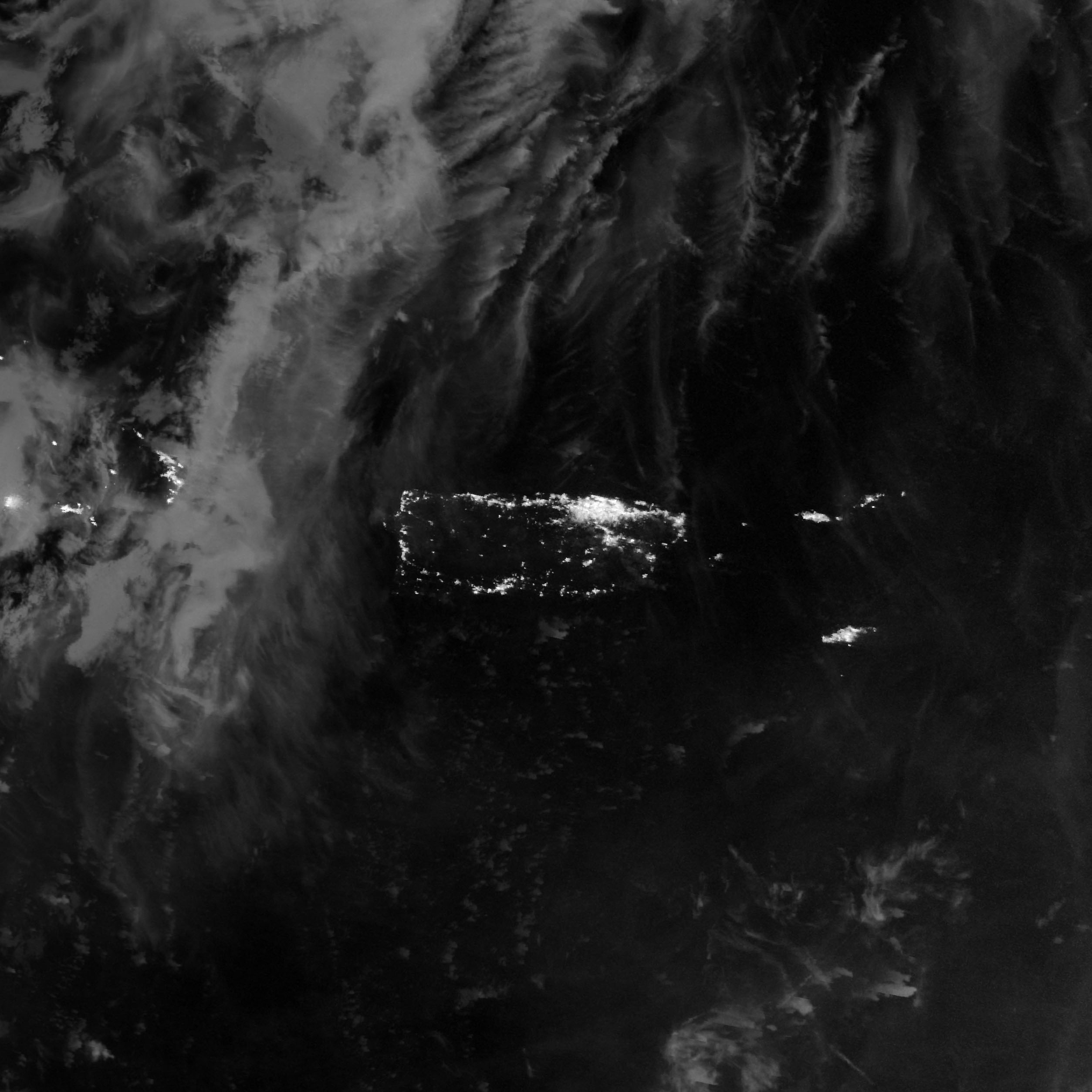This black and white photograph appears to have been taken from a high altitude, possibly even a satellite image from space. The image captures a sprawling city at night, with countless bright white dots illustrating the lights from buildings and streets. The city itself is outlined in a large, somewhat oval shape, with a densely lit downtown area at its center. Surrounding this central hub are more scattered lights, indicating the suburbs and shopping areas. To the left of the image, thin white clouds float over the surface, adding to the ethereal quality of the photograph. Small islands, also dotted with lights, can be seen around the main city, contributing to the intricate and mesmerizing nightscape. The overall scene is reminiscent of an island viewed from space, surrounded by dark waters, giving an almost mystical feel to the captured landscape.